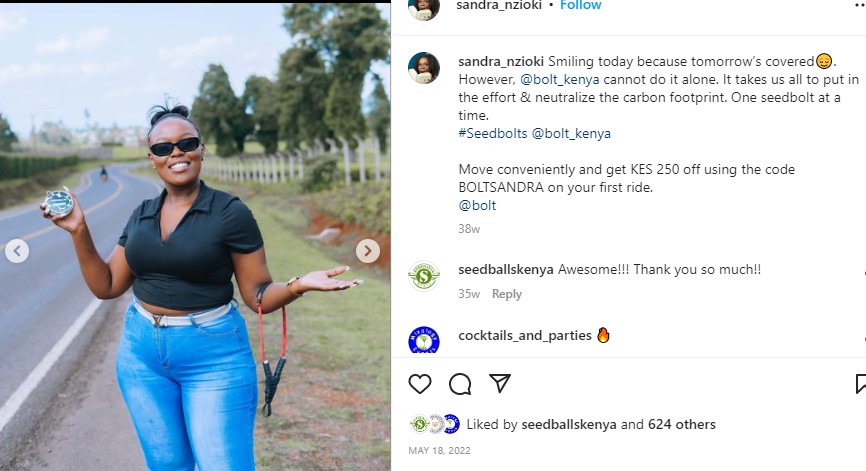In this wide rectangular Instagram post, the left half showcases a tall photograph of a black woman posing confidently by the side of a two-lane paved road. The road is marked with yellow and white paint and stretches into the horizon. The woman, identified as Sandra Zioki, has light brown skin and is adorned in a cropped black polo shirt, black sunglasses, and blue jeans cinched with a white belt. Her dark hair is styled in a ponytail, and she is smiling brightly, revealing white teeth. Both of her arms are raised; her right hand holds a round black object, and a red rope drapes over her left elbow. Behind her, there’s a lush backdrop of tall dark green trees, a white fence, grass, bushes, and a distant white building. A cyclist can be seen riding down the street. To the right of the photo is a caption that reads, "Smiling today because tomorrow's covered. However, at Bolt Kenya, we cannot do it alone. It takes all of us to put in the effort and neutralize the carbon footprint, one seed bolt at a time. #SeedBoltsAtBoltKenya. Move conveniently and get KES 250 off using the code BoltSandra on your first ride at Bolt." Below the caption are comments, including one from "Bolt Kenya" saying "Awesome," and another from "Cocktails and Parties" featuring a fire emoji. The post, dated May 18, 2022, also provides options to like, comment, or share.